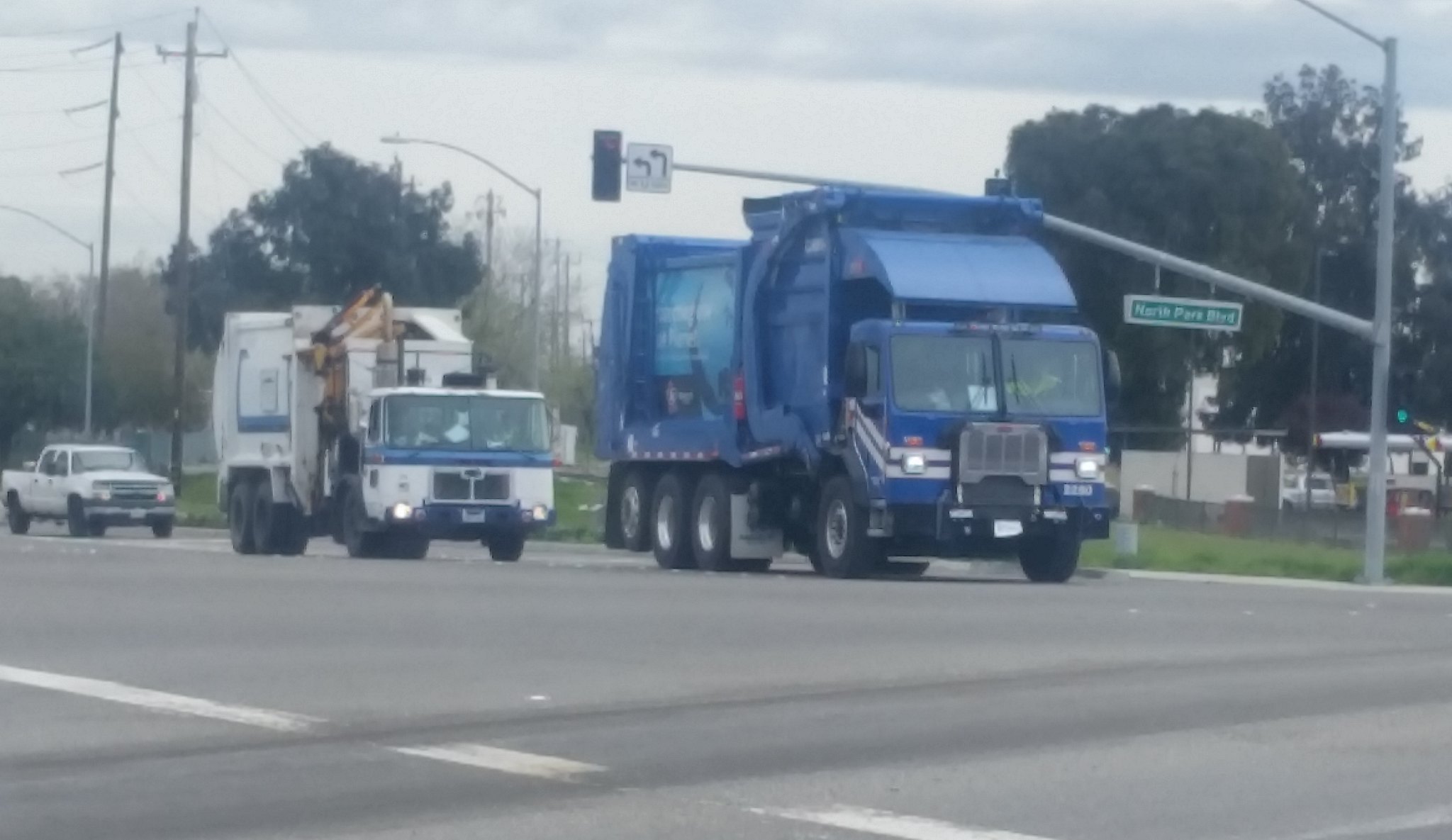The image captures a busy street intersection under a cloudy sky. Dominating the foreground is a large blue garbage truck, distinguished by its royal blue color and white stripes across its cab. This truck, equipped with ten wheels and a prominent grill, waits at a red light located under a street light and a left turn signal. Close behind, there is a white utility truck adorned with blue trim, also featuring ten wheels. Further back, a white pickup truck with an extended cab and four wheels is visible.

Surrounding the intersection, one can observe several power poles with power lines crisscrossing above. A tall street light rises in the center background, amidst a line of dark green trees. To the right side of the image, construction activities are apparent. The street, labeled as North Park Boulevard on a green sign with white text, is dark gray with white markings. Adjacent to the boulevard sign, a metallic pole extends a traffic light and a directional arrow into the scene.